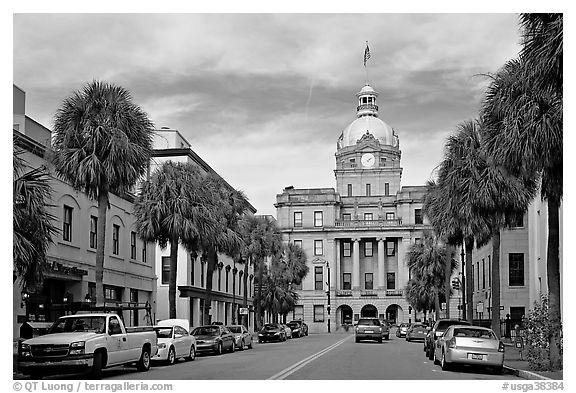In this black-and-white photograph, the view is from street level, looking down a city street towards a prominent, multi-story stone building that appears to be a town hall or courthouse. The imposing structure boasts a colonial architectural style, topped with a smaller story that features a clock face, a dome with a cupola, and an American flag waving from a flagpole. Flanking the street are tall, tropical-like palm trees, with approximately six on each side, their branches elegantly curving downwards. The street is lined with a series of parked cars ranging from pickup trucks to sedans, suggesting the image captures a scene from the 80s, 90s, or early 2000s. There are also a couple of vehicles, including an SUV or a wagon, cruising towards the central building. The buildings on either side of the street are two to three stories tall, adding to the urban landscape. The sky above is partly cloudy, with a hint of sunlight casting a soft glow, and a potential strike of lightning can be seen in the background to the left of the central building.